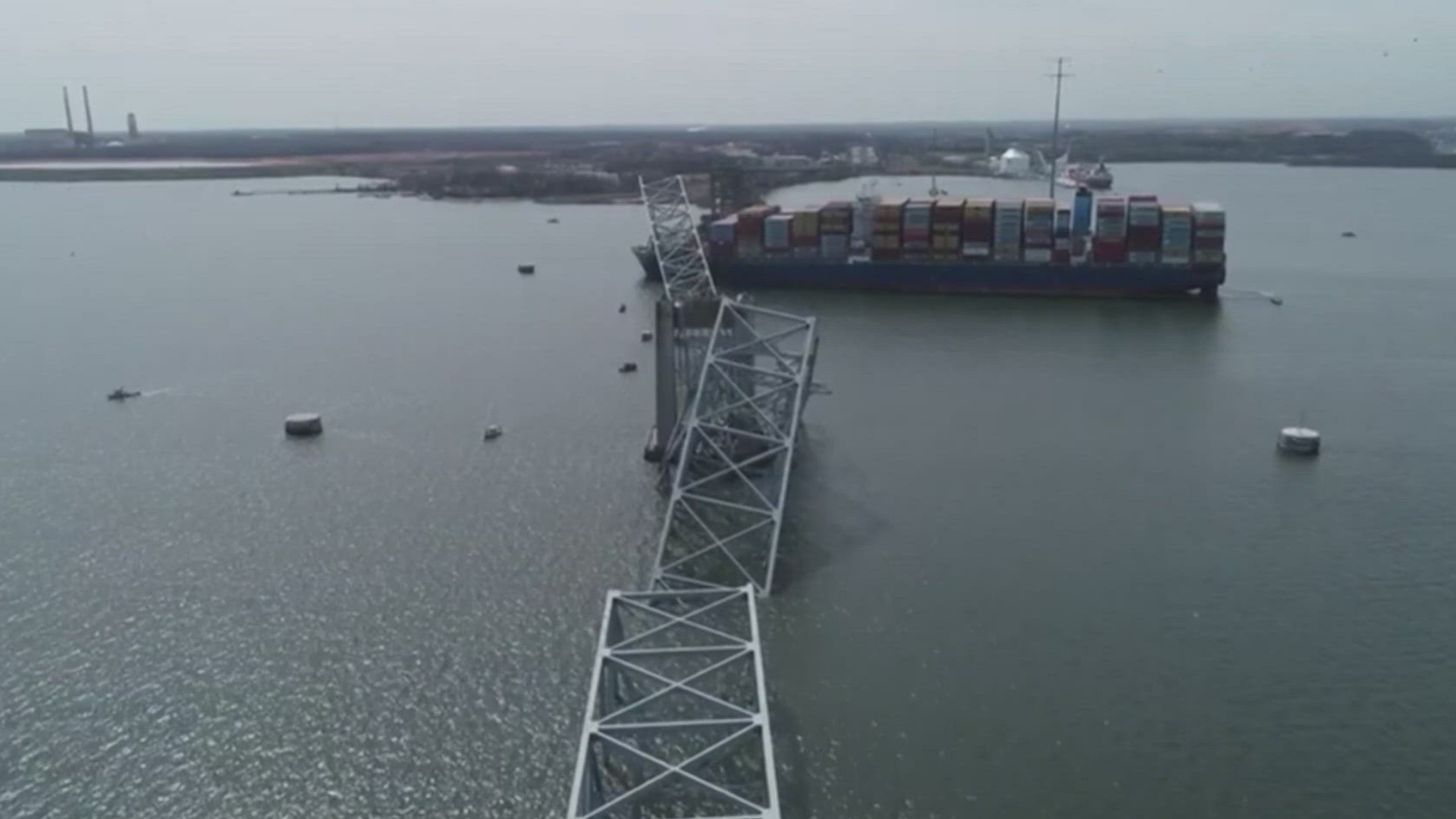The photograph captures a dramatic scene of a recent container ship collision with a bridge, likely in New Jersey. The image, possibly taken from a helicopter, showcases a cloudy gray sky as the backdrop. Just below the sky, a strip of land extends horizontally with a few power lines and distant buildings visible. Dominating the center of the image is the collapsed bridge, characterized by its metal supports with X-shaped patterns and square segments. The bridge is seen in disarray, with sections submerged in the gray water and others tilted upward. The large blue container ship with a reddish hull has plowed into the bridge, causing the structure to crumble into the river. The ship's deck is lined with numerous cargo containers. Additionally, various objects, possibly debris from the bridge, float in the water, accompanied by a few smaller boats navigating the area.